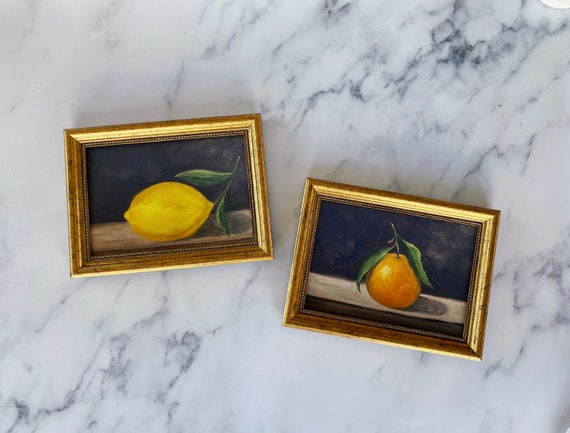This detailed color photograph showcases two framed paintings of fruit displayed on a predominantly white marble surface with subtle black streaks. Each painting is housed in a gold frame and features a black background. On the left, there is a realistic depiction of a lemon, complete with two green leaves attached to its stem. The vibrant yellow lemon rests on a light tan surface, providing a striking contrast to the background. On the right, a similar painting portrays an orange with a pair of green leaves sprouting from its stem. Like the lemon, the orange is set against the same kind of blue and light tan surface. Both paintings are arranged flat on the marble surface, capturing the detailed textures and colors of the fruit, and adding depth with subtle reflections cast on the tan surfaces they sit upon.